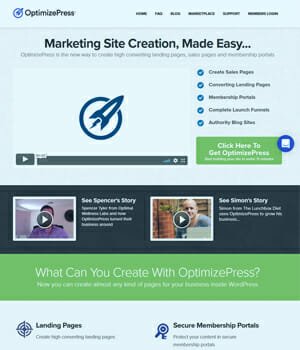This is an image from the homepage of the Optimize Press website. Dominating the main frame is the prominent caption, "Marketing Site Creation Made Easy." Below this headline is a large rectangular box designated for a video file, with a play button located at the bottom left corner.

The website's logo, an outline of a rocket ship set against a circle, is visibly displayed. To the right of the logo, there are five bullet points detailing the features of using the Optimize Press service.

Beneath the video box, two thumbnail images represent testimonials from users Spencer and Simon. These thumbnails can be clicked to view first-hand accounts of how Optimize Press has benefited their work.

Further down, a green background stripe contains white text that reads, "What Can You Create with Optimize Press?"